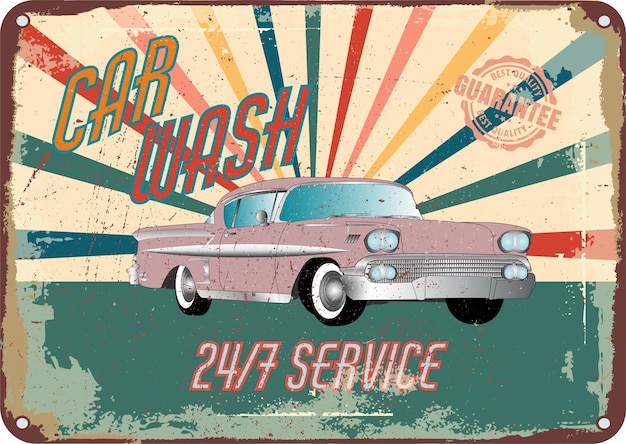This detailed image depicts a vintage 1950s-style metal advertisement sign for a car wash. In the center is an old pink car, likely a mid-1950s Chevrolet, possibly a Cadillac, drawn in a cartoonish style with white wall tires and headlights. Surrounding the car are vibrant, alternating rays of blue, green, red, pink, and yellow that mimic sunbeams. The upper left corner has the bold, stylized text "Car Wash" in orange and red 1950s-themed lettering. On the upper right is a circular stamp, the same mauve-pink color as the car, declaring "Best Quality Guarantee." Along the top and bottom of the circle, the text reads "Best Quality." Beneath the car, on a greenish-gray teal background, is a bold message announcing "24-7 Service." The sign shows signs of aging with rust around its edges and has four holes, suggesting it was once mounted.